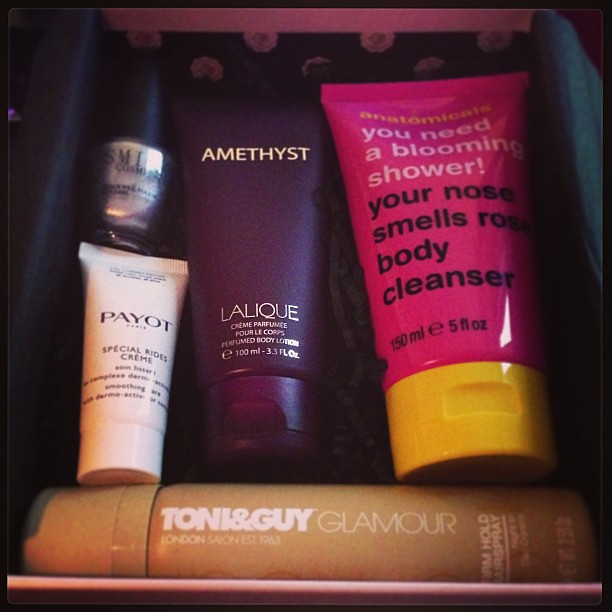This image is a detailed collection of various cosmetics displayed in an open box with a piece of black paper underneath. The box itself is pink on the sides. From left to right, the assortment includes:

- A small bottle of silver nail polish with a black cap and black text on its clear body.
- A white tube labeled "P-A-Y-O-T, special rides cream" in black text.
- A rich burgundy purple tube with "amethyst" in yellow text at the top and "LALIQUE" in white text towards the bottom, identified as a cream perfume.
- A bright hot pink tube with a yellow cap, which in yellow text says "anatomicals," in white text says, "you need a blooming shower," and in black text, "your nose smells rose, body cleanser."
- Along the bottom, there's a brown bottle with white text reading "Tony and Guy Glamour London Salon firm hold hairspray."

This assortment consists of four tubes and one nail polish bottle, showcasing a variety of beauty products in an attractive and organized manner.